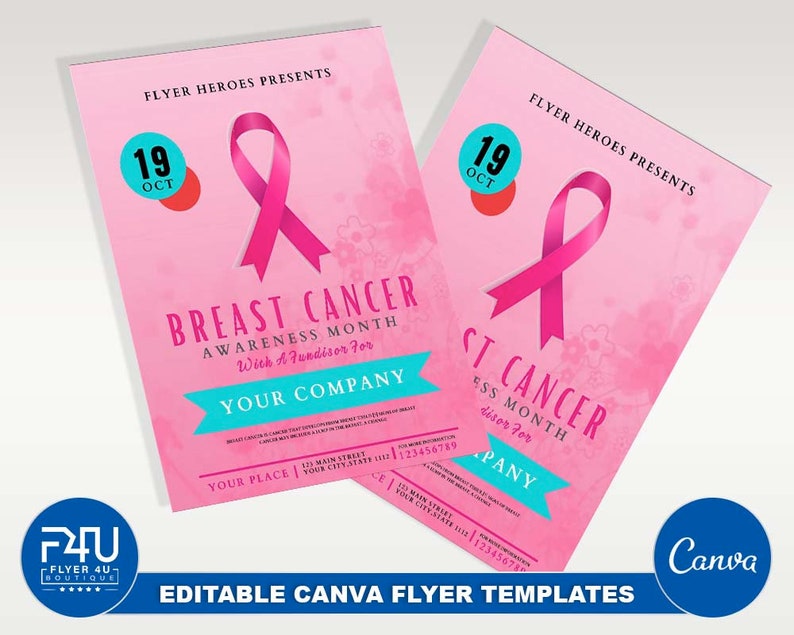The image features two pamphlets placed on an off-white background, with one pamphlet slightly overlapping the other. Both pamphlets display identical content. They have a vibrant pink background with the headline "Flyer Heroes Presents." Central to the design is a prominent pink ribbon symbol for breast cancer awareness. To the left of the ribbon, a blue circle contains the date "19th of October."

Below the ribbon, the text reads "Breast Cancer Awareness Month" followed by a segment indicating a fundraiser, which prominently displays the placeholder text "Your Company" within a blue banner. A small section of black text is situated below this banner; however, it is illegible.

At the pamphlet's bottom, the location details are provided: "Your Place, 123 Main Street, Your City, State," accompanied by a generic phone number, "123456789." The base of the flyer features a blue banner with decorative blue circles on either end. The left circle contains the text "FV4U, Flyer4U Boutique, 5 Stars," while the right circle features the Canva logo. Spanning across the blue banner in white text is the phrase "Editable Canva Flyer Templates."

The detailed and organized layout effectively conveys crucial information about a breast cancer awareness event, combining a clean design with strategic color usage for a visually appealing and informative pamphlet.